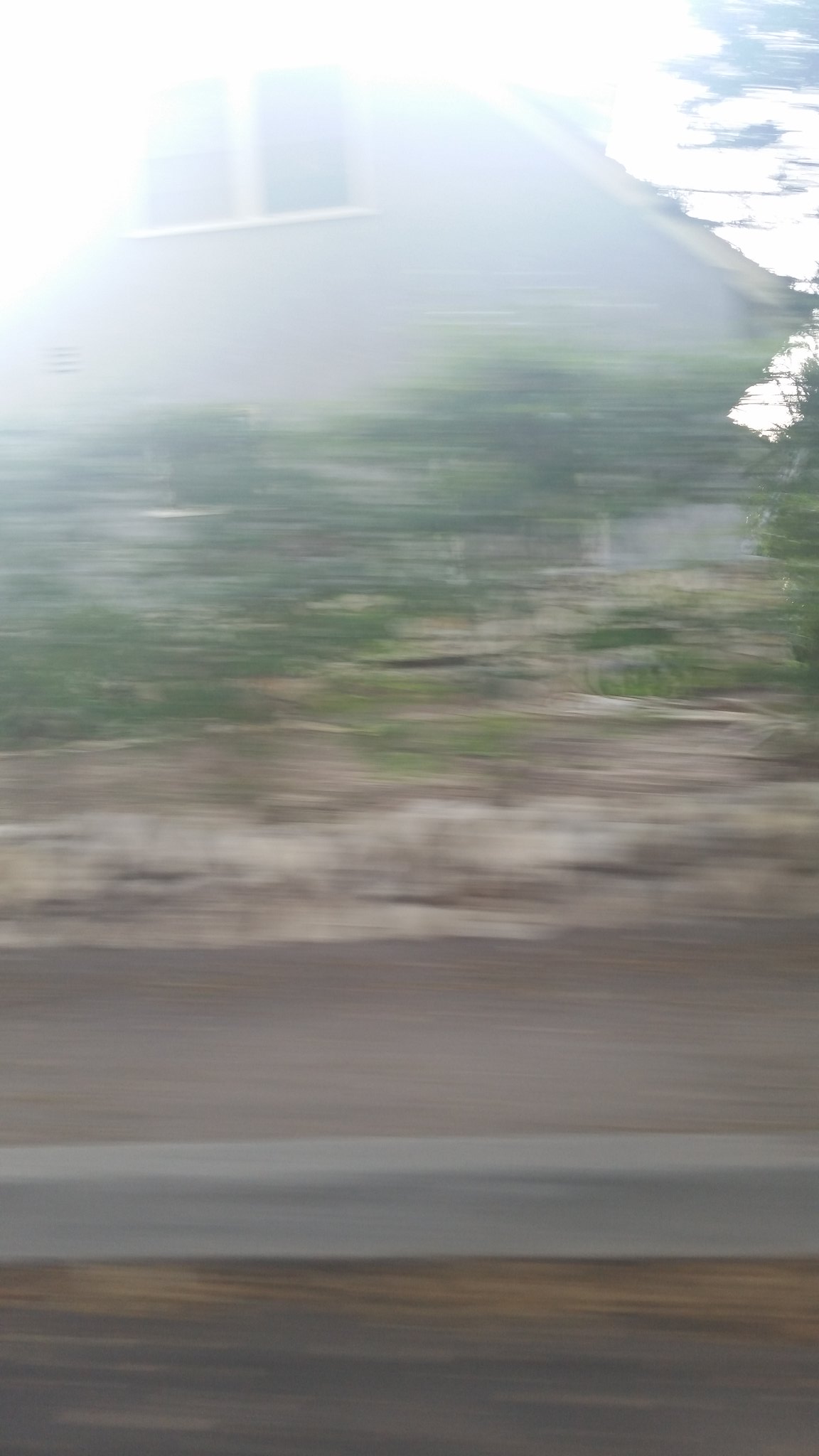This image appears to be a photograph likely taken from a moving car, resulting in a significant motion blur. The photograph features a gray house prominently displayed in the hazy background, with a noticeable window at the top left. The lighting at the top of the image seems almost excessively bright, contributing to the overexposed, washed-out appearance. The house features a window with a white frame divided into two panels. Below the house, the scene transitions into a grassy area followed by a strip of dirt and a concrete wall. Alongside the road, a long horizontal metal railing is visible. The top left corner of the image is marked by a bright light source, adding to the overall blurry and hazy aesthetic of the photograph.